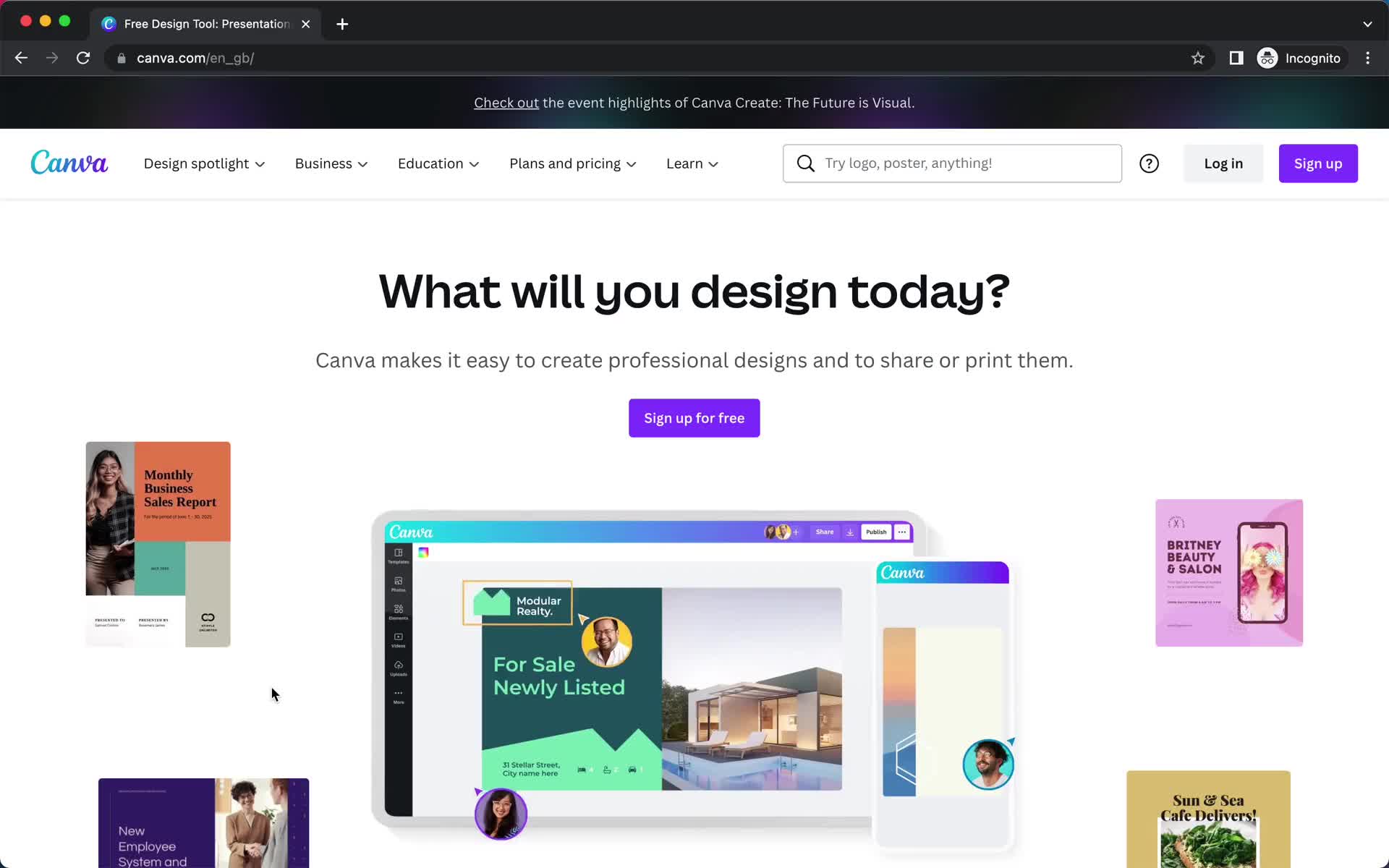This is a detailed annotated screenshot of the Canva website as viewed in a dark-themed web browser. At the top center of the site, there's a banner that reads, "Check out the event highlights of Canva" followed by "Create the future of JizzleRoll" and the Canva logo. Below the banner, there are navigational tabs labeled: "Design Spotlight," "Denaro," "Business," "Denaro," "Education," "Denaro," "Plans and Prices," "Denaro," "Learn," "Class," "Class," "Try," "Logs," "Logo," "Poster," and more. Additionally, there are options to "Login" or "Sign up."

Beneath the navigation tabs, a prominent text invites users to "sign up to design today," asserting that "Canva makes it easy to create professional designs and to share them." A distinct "Sign up for free" button is positioned centrally.

To the left, an image depicts a brochure titled "Monthly Business Sales Report" featuring a smiling woman. Below it, another brochure reads "New Employee System," also with a smiling woman.

To the right of these brochures, there's a detailed screenshot showcasing Canva's interface in use for creating a "For Sale Newly Listed House" flyer. Further right, another screenshot displays Canva accessed via a mobile phone.

Adjacent to these, a brochure titled "Brittany Beauty and Salon," featuring a woman on the phone, is visible. Underneath this, a flyer announces "Someone's Cafe Delivers."